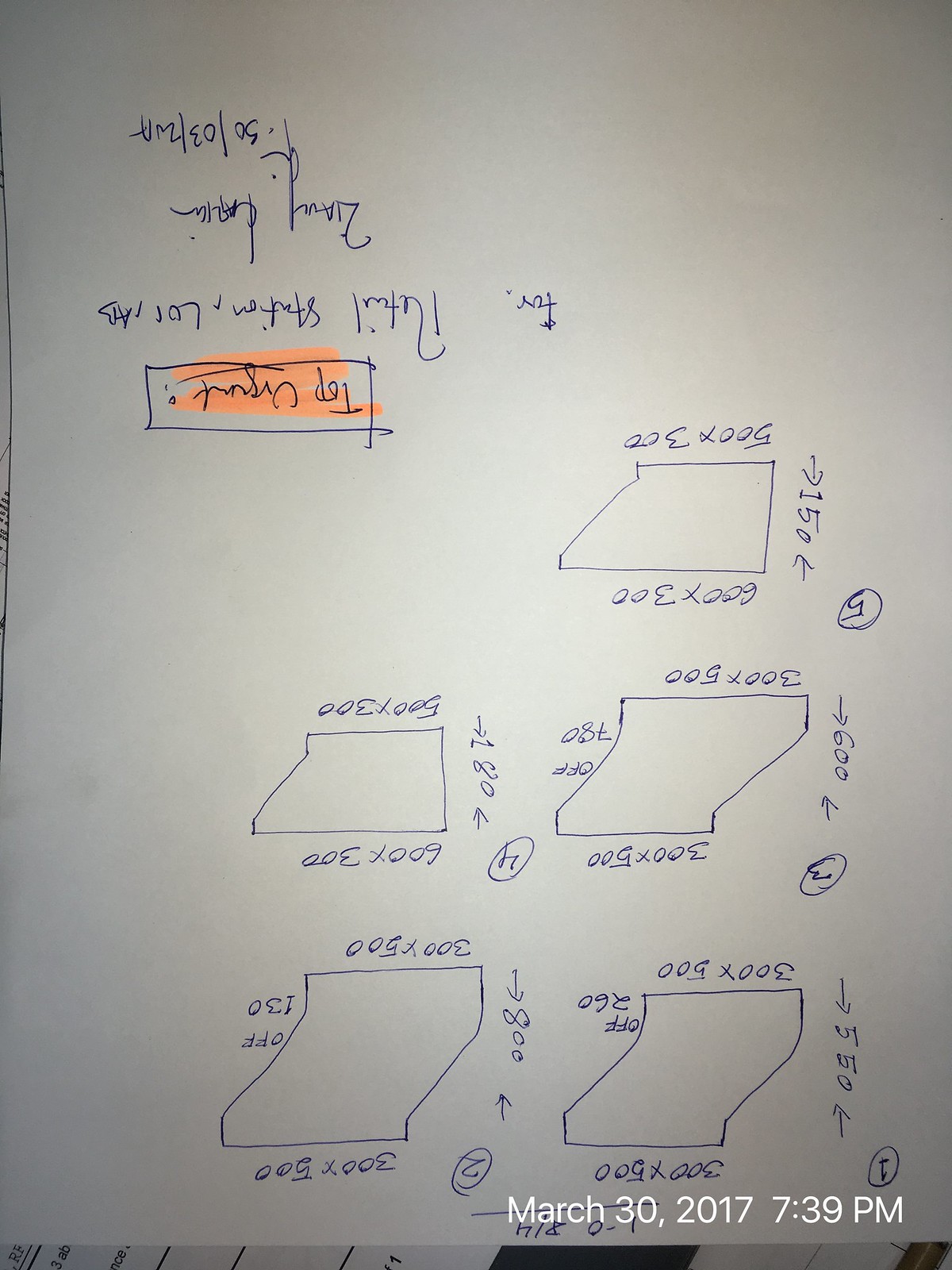This is a photograph of an upside-down white piece of paper with the date and time "March 30th, 2017, 7:39 p.m." written in white in the bottom right-hand corner. The paper features a hand-drawn diagram consisting of five figures arranged in a grid. These figures are not quite square but are labeled 1 through 5. Their positions are as follows: 

1 is at the top left, 
2 is next to 1 on the top row, 
3 is directly below 1,
4 is directly below 2, 
5 is directly below 3.

Each figure includes dimensions written horizontally on top and below, as well as vertically oriented height measurements written on the left-hand side:

- Figure 1: 300 by 500 (Top and Bottom), height 550.
- Figure 2: 300 by 500 (Top and Bottom), height 800.
- Figure 3: 300 by 500 (Top and Bottom), height 600.
- Figure 4: 600 by 300 (Top), 500 by 300 (Bottom), height 180.
- Figure 5: 600 by 300 (Top), 500 by 300 (Bottom), height 150.

In the bottom right-hand corner of the document, there is a highlighted box with the text "Top Urgent" marked in orange. Below this is another note that appears to be for a retail station lot, though the full text is illegible, possibly reading "L-O-R, A-B." Following that, there is a seemingly handwritten name that is difficult to decipher but looks like “2-I-A-V-Y” followed by “Carrion” and the date "30-03-2017."

This detailed illustration seems to be depicting various design options with specific dimensions, perhaps for some sort of planning or architectural purpose. The upside-down orientation and faint handwriting make the information challenging to read.